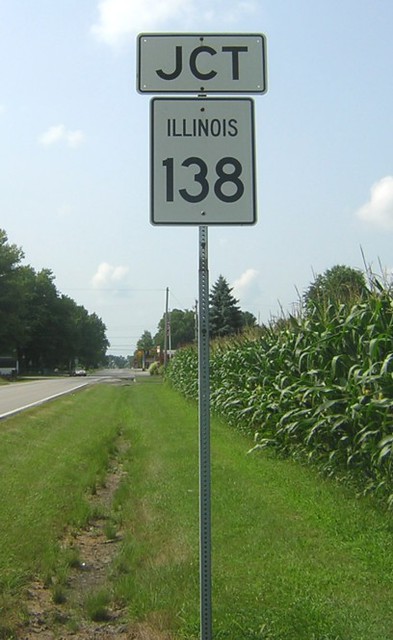This vertically-oriented color photograph captures a picturesque roadside scene on a sunny day. The image is taken beside a slight ditch that runs parallel to a grassy area, with patches of dirt visible in the bottom left corner. Dominating the center of the photo is a thin metal street sign, consisting of two sections: a white rectangular sign with black text reading "JCT" on top, and below it, a vertical rectangle signifying "Illinois 138." To the right, expansive cornfields stretch out, contributing to a sense of rural tranquility. The photograph's perspective draws the viewer's eye back towards a vanishing point, emphasizing the depth of the scene. On the left side of the image, a road runs adjacent to the grassy strip, lined with a row of trees that adds a natural frame to the composition. The sky is a brilliant, light blue with a scattering of fluffy white clouds, creating an idyllic backdrop to this quintessential Midwestern landscape.